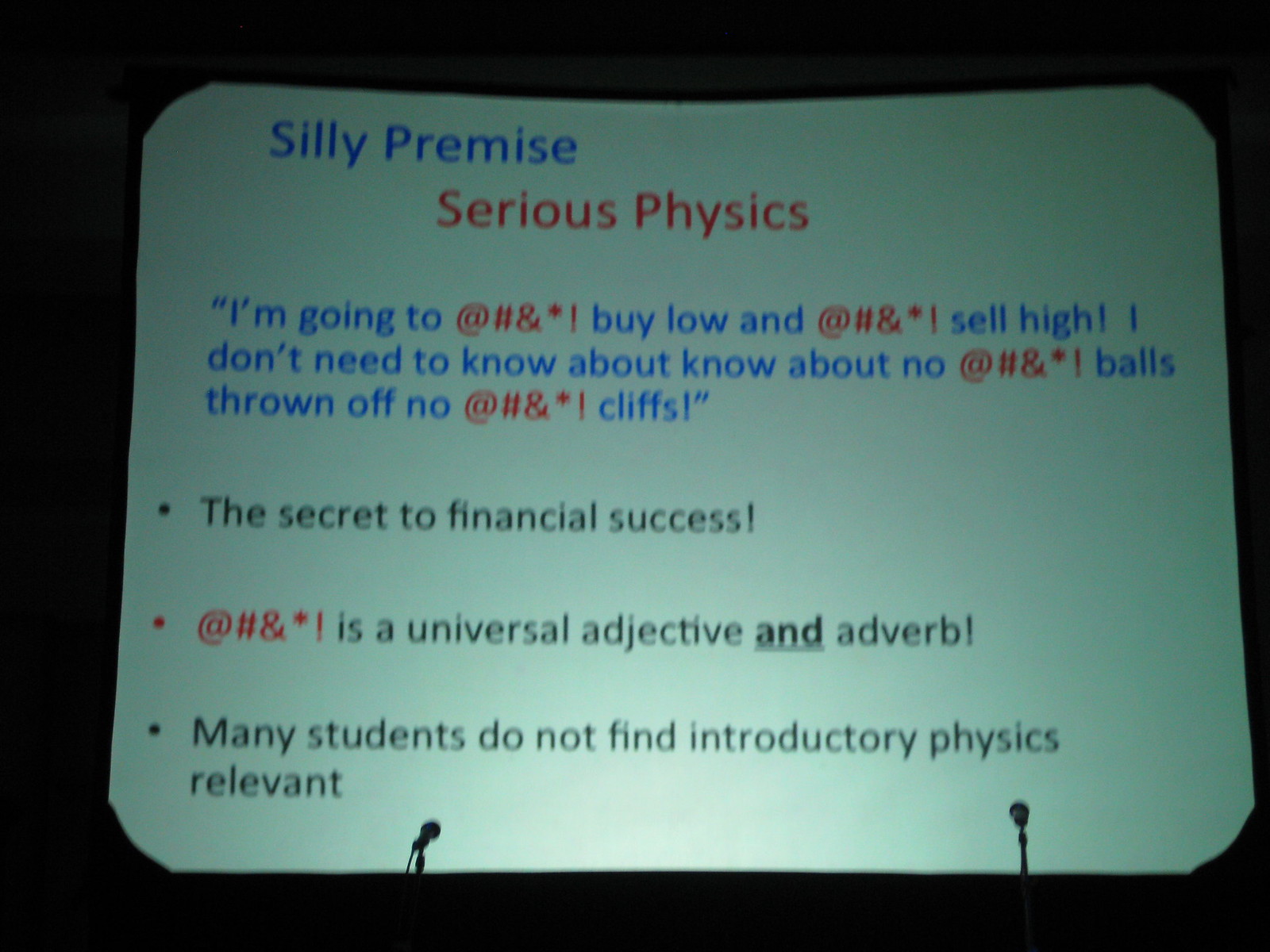The image presents a projected screen set against a black background during an indoor presentation. Central to the image is a white screen with text in various colors: blue, red, and black. At the bottom of the screen, two microphone stands are visible on either side. The screen's text begins with "Silly premise, serious physics" in blue and red at the top. Below, a quote in blue text with segments censored by red symbols (e.g., @, #, &, *, !) reads: "I'm going to bleep by low and bleep sell high. I don't need to know about no bleep balls thrown off no bleep cliffs." Further down are three bullet points in black text: "The secret to financial success," followed by, "bleep is a universal adjective and adverb," and concluding with, "Many students do not find introductory physics relevant." The setting and style suggest a formal presentation focused on making physics education engaging.